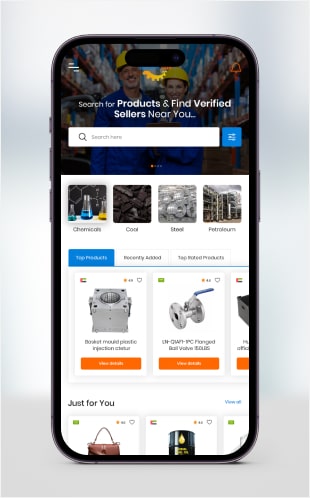A detailed photograph showcases a smartphone lying on a sleek gray background. On the phone's screen, a user interface prompts the user with the text, "Search for products and find verified sellers near you." The backdrop of the phone's display features an image of two individuals wearing hard hats inside a large warehouse with shelves stocked high with various items. The search bar, highlighted in white, invites users to "search here." Below the search bar, categories such as "Chemicals," "Coal," "Stools," and "Petroleum" are listed. Furthermore, featured top products include an image of a production bucket and a mold for plastic injection, as well as a valve visible next to them. Additionally, a section labeled "Just for You" displays a purse and what appears to be a candle, though partially obscured.